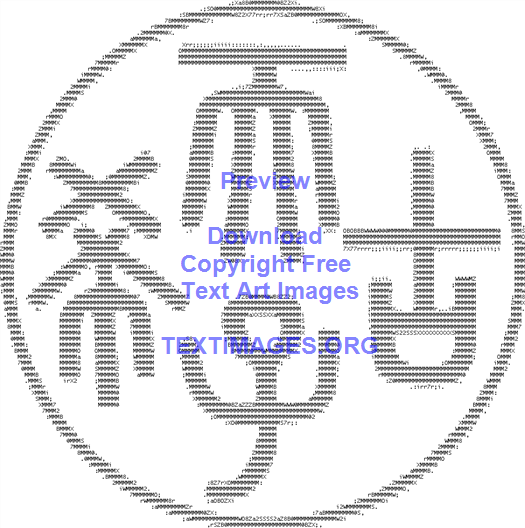This digital artwork is composed of numerous small black numbers and letters intricately organized to form an elaborate pattern. At the center of this pattern is a prominent circle, within which four distinct shapes or characters are positioned at the top, bottom, left, and right. These characters bear a resemblance to Chinese or Japanese symbols but are intricately crafted from rows of various letters and numbers, giving the impression of an image created through coding. The overall design is set against a white background, and overlaid at the top is a periwinkle blue text that reads "preview, download, copyright-free, text art images, textimages.org". The image showcases a clever use of typography and digital art principles to create a visually captivating representation.